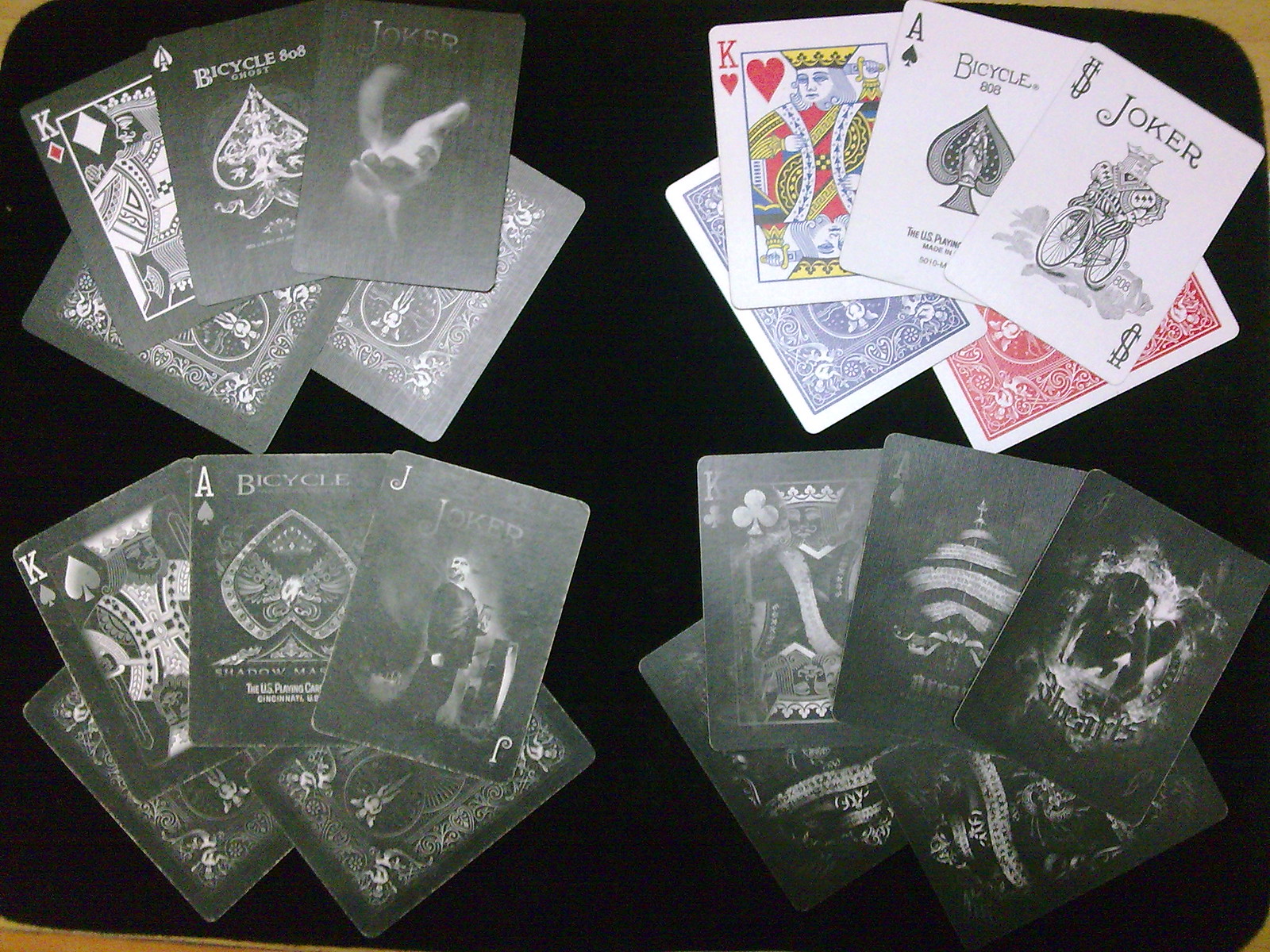The photograph captures a top-down view of four sets of playing cards, each with their unique decorative styles.

In the upper right-hand corner, the set features traditional Bicycle-branded cards. The card on the right is a Joker, marked with "Bicycle 808". It showcases a traditional design with the word "JOKER" in a classic font at the top and a symbol reminiscent of a dollar sign in the corners. The illustration on the Joker card depicts a king riding a bicycle. To the left of the Joker is a King of Hearts card, displaying a conventional red and blue decorative design.

The upper left-hand corner set consists of Bicycle Ghost cards. The King of Diamonds in this set is accompanied by a ghostly-themed Joker card, featuring an eerie hand reaching out.

In the bottom left, the Bicycle Shadow Master set is presented. It includes a King, an Ace, a Jack, and another Joker card, characterized by a black and smoky gray color scheme. The Joker in this set is represented by a prominent "J" in the corners and an illustration of a man bending backward.

The final set, located in the bottom right, also follows a black and smoky gray theme. It features a King, an Ace, and a Joker card. This Joker card is particularly striking, depicting a woman crawling through flames, and it intriguingly displays "Three Hearts" on the card.

Each set brings a distinct aesthetic, combining traditional and modern, eerie elements.